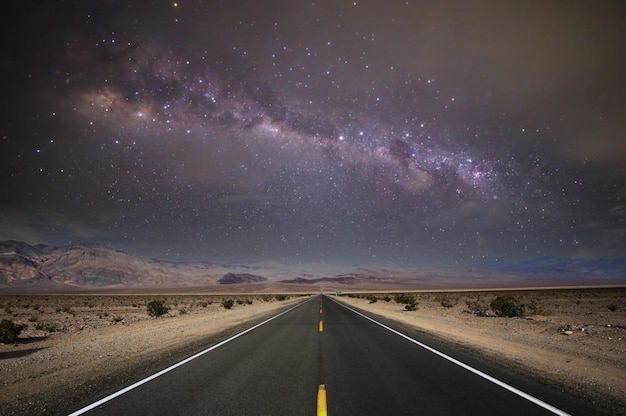In this color photograph taken from the center of a lengthy and straight two-lane asphalt highway, the perspective stretches off directly into the distant horizon beneath a night sky. The road features dashed yellow lines down the center and solid white lines along the edges, with sandy dirt shoulders flanking each side. Surrounding the road is a barren desert landscape dotted with sparse, scrubby green bushes. In the distance, a rugged mountain range spans the background, with one particular mountain appearing flat on its far right side. 

Above, the night sky is richly detailed, showcasing the Milky Way in all its splendor. The sky is filled with clusters of stars forming a luminous band across the center, accompanied by light gray clouds scattered throughout. Some clouds exhibit a gaseous purple and gray hue, with glowing lights within them, while countless tiny white specks of stars twinkle across the dark expanse. Captured with apparent long exposure or post-processing enhancement, the image juxtaposes the desolate, lonely highway against the breathtaking, celestial beauty of the night sky, creating a striking and evocative scene.